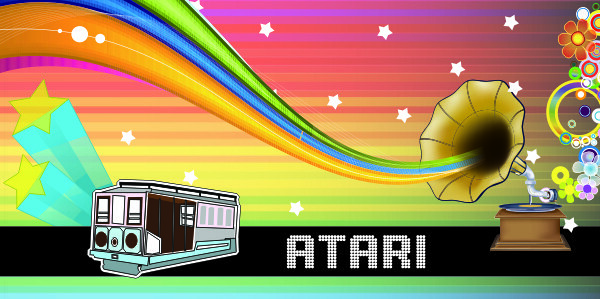The image is a vibrantly colored digital poster with a rectangular orientation, displaying a rainbow gradient background that transitions from darker reds at the top to lighter greens at the bottom in horizontal streaks. Dominating the right side of the image is an old-fashioned phonograph with a brass horn pointing left. A rainbow stream emerges from the horn, arching downward in the center before swooping up and out of the frame in the upper left. Situated at the bottom, a black strip spans the width of the poster, containing the pixelated, capitalized word "ATARI" in white letters. To the left of this text, there's a simple, three-quarter view depiction of a street trolley featuring a blue base, a light gray top, and pinkish accents. Sprinkled across the background are approximately 10 to 12 small, randomly spaced stars. In the upper right corner, various multicolored floral circles add a whimsical touch to the composition.